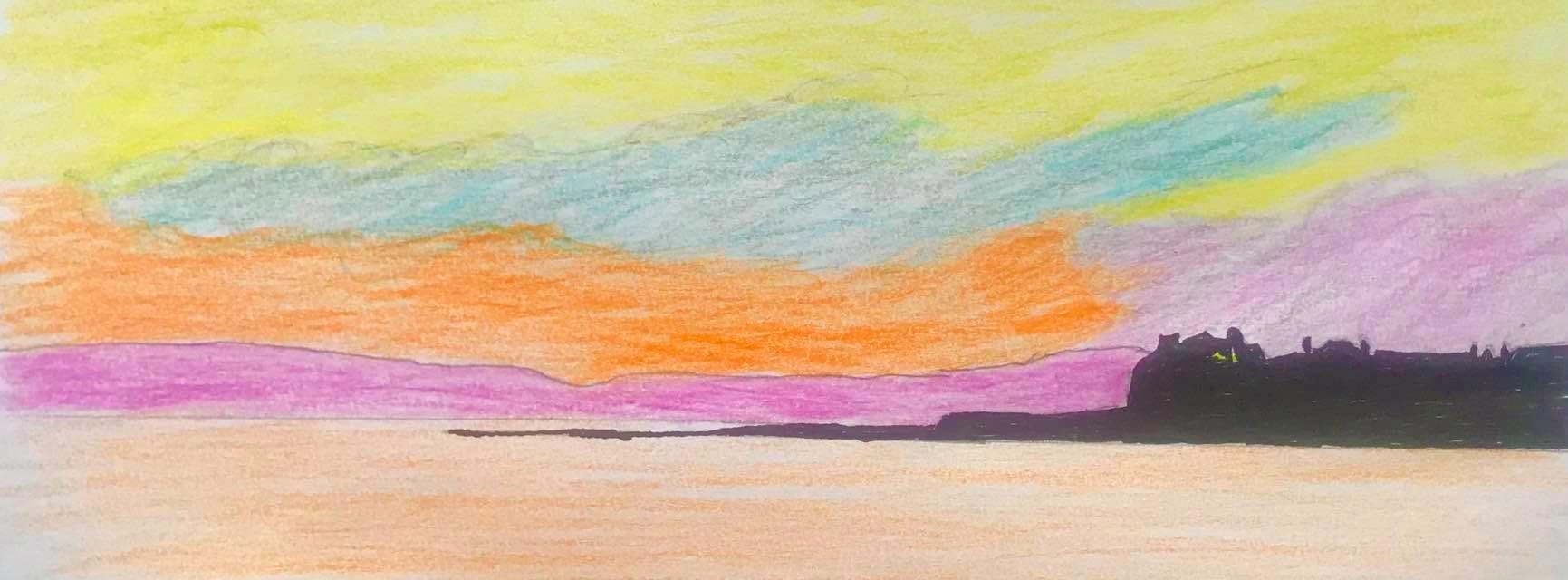This drawing depicts a unique and vibrant landscape. The water is colored a striking orange, creating an unusual yet captivating scene. To the far right, there is a mass of black which appears to represent land, possibly featuring indistinct structures silhouetted against the sky. Above the water and adjacent to the land, a patch of pink ground contrasts vividly. The sky transitions through a spectrum of colors: orange on the left, fading into pink, followed by a section of blue that appears cloud-like, and finally culminating in a broad expanse of yellow at the top. The artwork, seemingly crafted with crayons, exhibits a scribbled texture with discernible pencil lines adding subtle detail and depth.